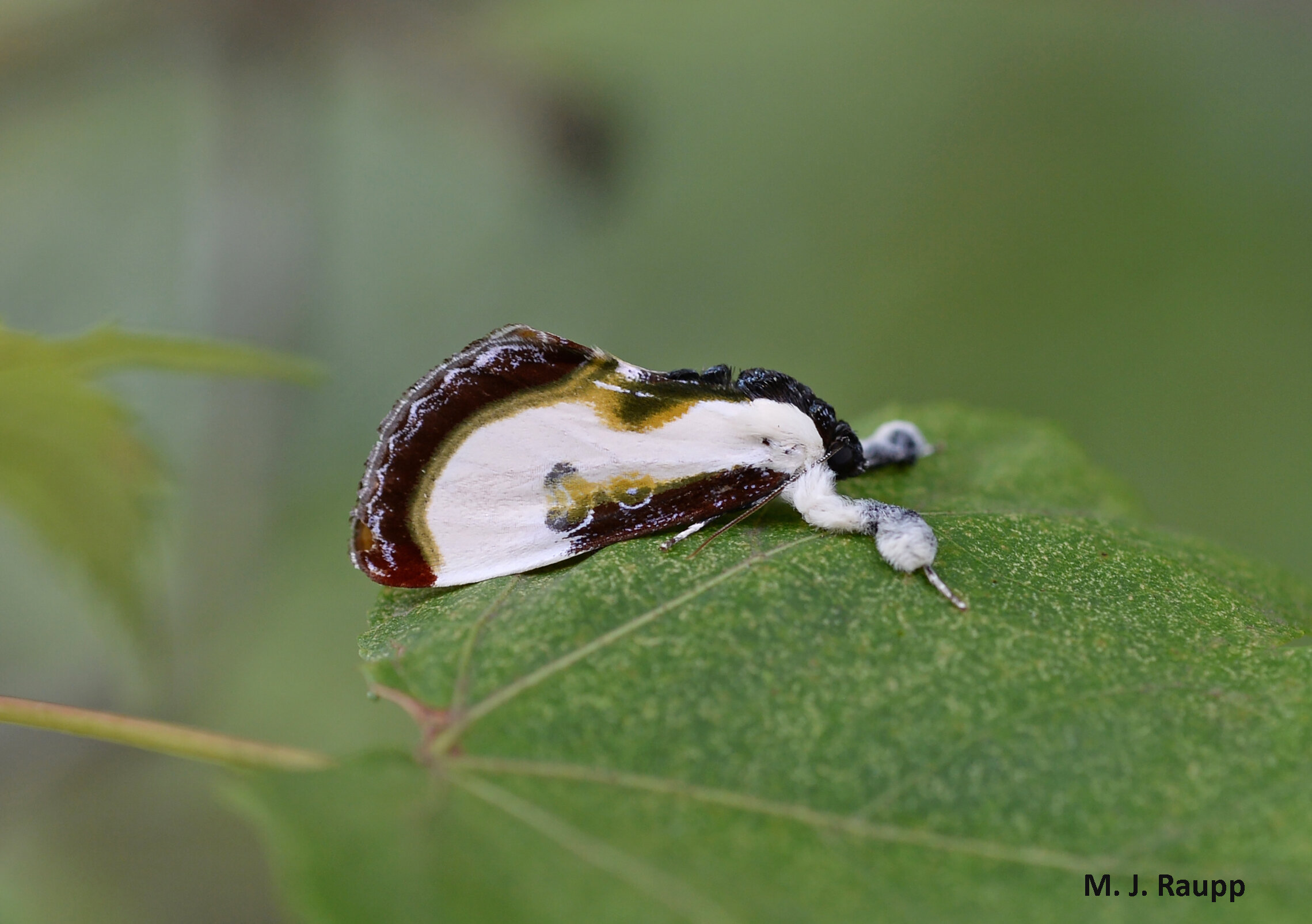The outdoor photograph is a close-up of an enigmatic insect perched on a green leaf, its identity sparking debate. The creature's peculiar form, possibly a moth or butterfly, features a white wing bordered in brown and accented with hues of greenish-yellow and black. Notably, the wing is marked by two distinctive black spots. Adding to its odd appearance, the insect has limb-like structures that resemble a beak protruding from a goose or duck-like head, which further confounds its identification. The overall composition renders the leaf's veins in a contrasting light green, set against a softly blurred, grayish backdrop. In the bottom right corner, the text "MJ are you APP" is inscribed in black.